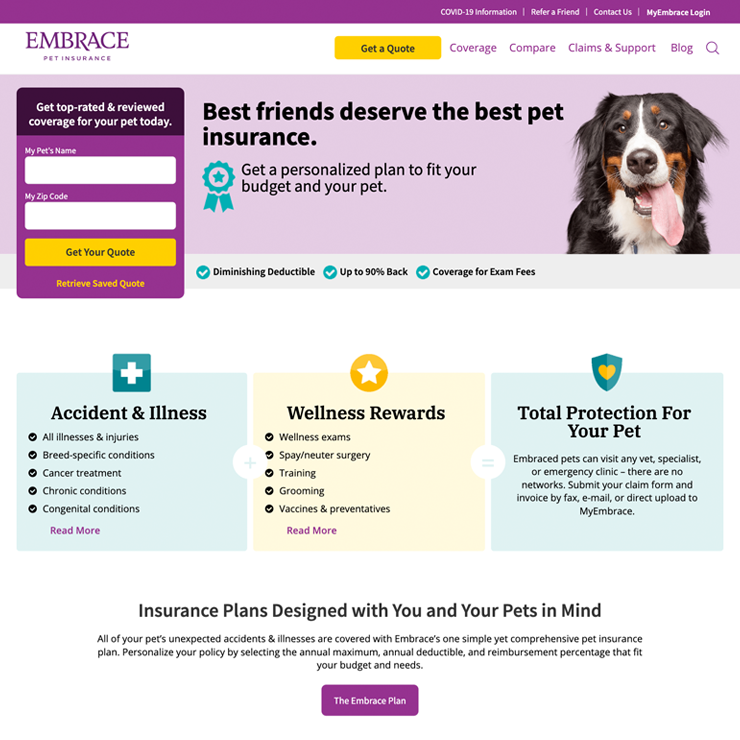The homepage of the Embrace Pet Insurance website features a vibrant and inviting design characterized by a palette of light purple, dark purple, yellow, blue, black, brown, and pink colors. Dominating the top section of the page is a heartwarming image of a tri-colored dog with black, brown, and white fur. The dog's tongue is playfully hanging out as it looks straight ahead, adding a friendly touch to the page. 

The header prominently displays "Embrace Pet Insurance" alongside a yellow rectangular button that invites visitors to "Get a Quote." Above this, navigation links are available for COVID-19 information, referring a friend, contacting the company, and logging into the "My Embrace" account. 

Adjacent to the quote button, additional links offer easy access to pages such as Coverage, Compare, Claims and Support, and the Blog. Just below the image of the dog, a slogan reads, "Best friends deserve the best pet insurance," accompanied by a small icon resembling an award. Another prompt encourages users to "Get a personalized plan to fit your budget and your pet."

On the left side, there is an input box for pet owners to enter their pet's name and zip code, accompanied by another yellow button to click for a quote. Beneath this section, three informational boxes provide details on the types of plans available: Accident & Illness, Wellness Rewards, and Total Protection for Your Pet. 

At the bottom of the homepage, a reassuring slogan states, "Insurance plans designed with you and your pet in mind," next to a purple button labeled "The Embrace Plan" that visitors can click for more information.